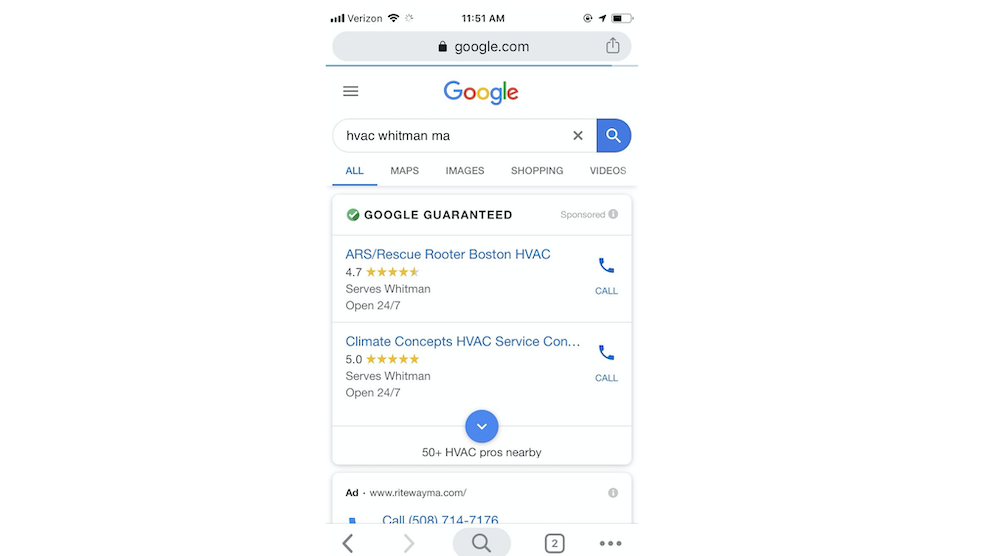The screenshot from a smartphone displays a variety of indicators and a Google search result page for HVAC services in Whitman, Massachusetts. 

Starting at the top left, the smartphone shows a strong Verizon carrier signal, followed by a full Wi-Fi signal, and a loading symbol. In the center, the current time reads "11:51 AM" in bold black text. Adjacent to the time, an almost completed circular loading icon with a smaller black circle and an arrow pointing right is visible. To the far right, there is a battery icon indicating approximately 25% charge remaining.

Below these status icons, there is a URL bar formatted as a gray oval with the text "google.com" accompanied by a lock symbol, indicating a secure site. To the right of the URL bar is a gray square with an upward arrow, suggesting an upload function.

The Google logo is located further below, consisting of a multicolored "G" followed by "oogle" in blue, red, yellow, and green respectively. To the left of the logo is a button with three horizontal lines indicating a menu or settings option.

Underneath the Google logo, there is a white oval search bar containing black text that reads "HVAC Whitman, MA." The search bar features a blue magnifying glass icon on the right end, along with an "X" for clearing the text.

Next, the webpage shows different tab options for the search, with "All" selected and highlighted in blue, followed by "Maps," "Images," "Shopping," and "Videos," which are in gray.

The main content displays a section labeled "Google Guaranteed" within a gray-bordered rectangle, offering a money-back guarantee for selected professionals. Below this are sponsored links: 

1. "ARS/Rescue Reuter Boston HVAC" with a phone icon for calling, showing a 4.7 out of 5 rating, serving Whitman, and available 24/7.
2. "Climate Control Concepts HVAC" with a blue truncated link and a perfect 5 out of 5 rating, also serving Whitman and open 24/7.

Below these sponsored links, there is a dark blue circle with a downward-pointing white arrow, labeled "50+ HVAC pros nearby" in black text.

At the very bottom, there is a partial view of another section with the label "Ad" in bold black font, alongside the website "www.rightwayma.com," and a call-to-action button with the text "(508) 714-7176" in a dark blue square. There is also a gray circle with a white "i" icon indicating more information.

Finally, the bottom navigation bar shows a back arrow in bold black, a gray forward arrow disabled, a dark gray circle with a black magnifying glass for searching, a square with a number "2" indicating two open windows, and three vertical ellipses for additional settings.

This comprehensive screenshot captures various elements of the phone's interface and the details of an ongoing search for HVAC services in Whitman, MA.